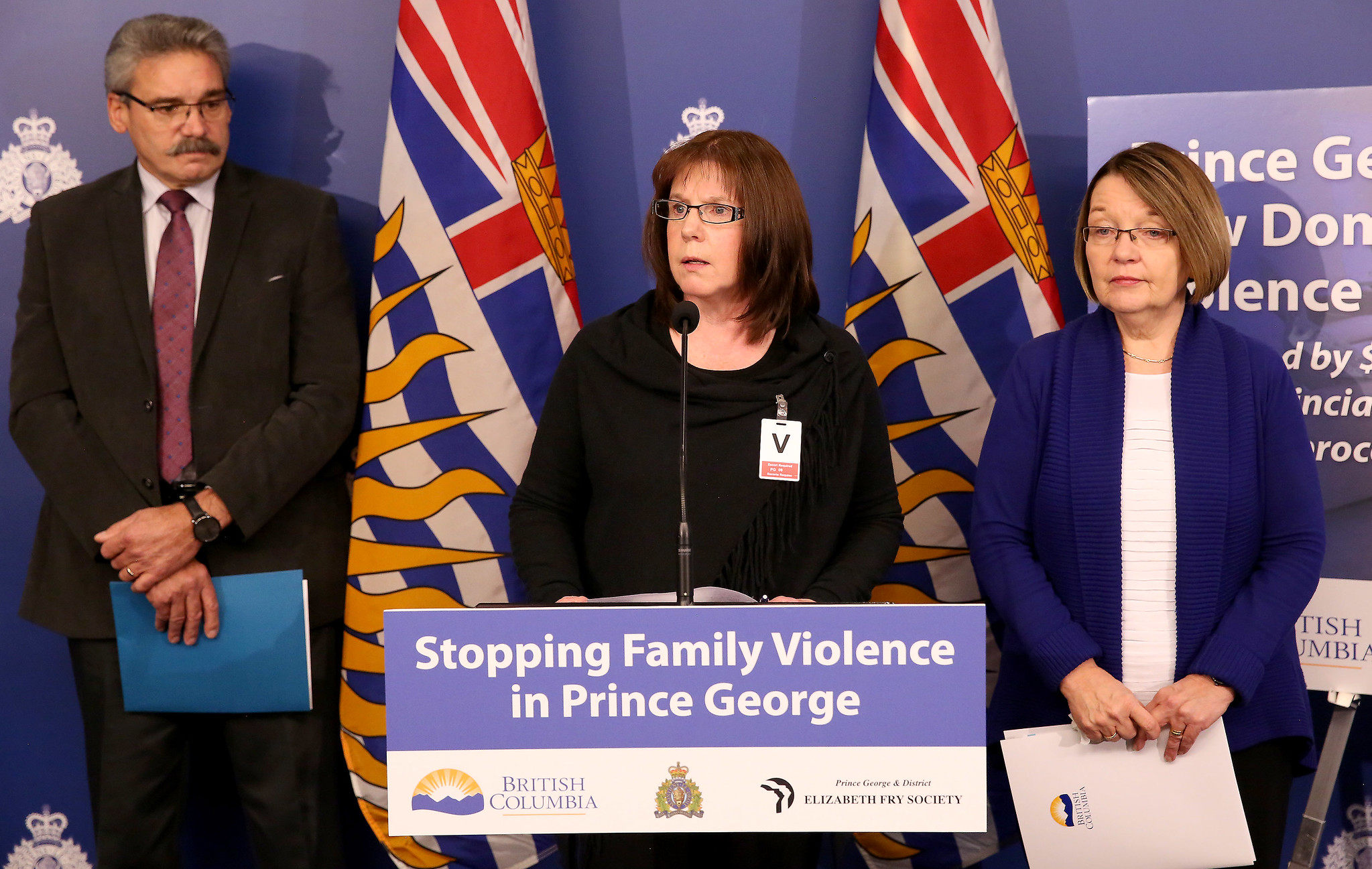The image depicts a press conference at a stage-setting podium with a sign that reads "Stopping Family Violence in Prince George," featuring the logos of British Columbia and the Elizabeth Fry Society. At the podium stands a middle-aged woman with straight, shoulder-length brown hair, wearing glasses, and a black shirt with a name tag bearing a large "V." To her left, there is an older man with graying hair and a mustache, dressed in a black suit and red tie, holding a blue folder. To her right, another middle-aged woman, wearing a blue sweater over a white blouse, stands with a serious expression, also holding notes. All three individuals, positioned in front of two national flags—presumably of British Columbia—appear serious and poised, signifying the event's sober tone focused on addressing family violence.